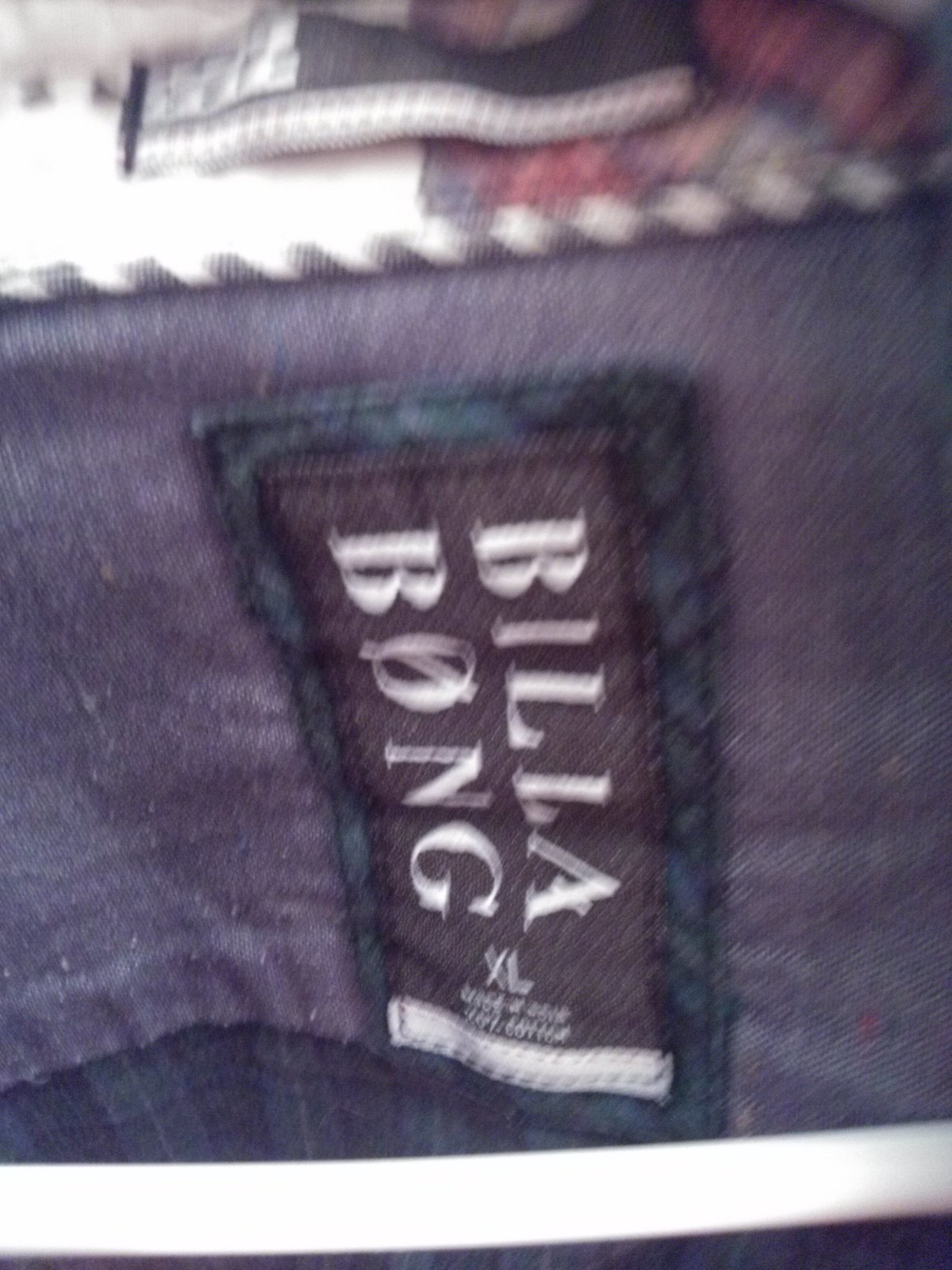This close-up image focuses on a clothing tag centered amidst the fabric. The prominent tag displays the brand "Billabong," known for its apparel, with an indication that the garment is an XL size. The surrounding material, though somewhat blurry, provides additional details. The upper portion of the fabric is a rich, jean-blue color, while the lower section transitions into a pattern resembling pajama bottoms. This pattern, comprised of rectangular squares, features a palette of dark blue, light blue, and dark green. The background behind the garment is indistinct, hinting at a carpet and a bit of flooring. The Billabong logo on the tag is oriented vertically, alongside the readout that the clothing is 100% cotton. Additionally, a white bar stretches horizontally across the fabric beneath the tag, its exact nature and purpose remaining unclear due to the blur.